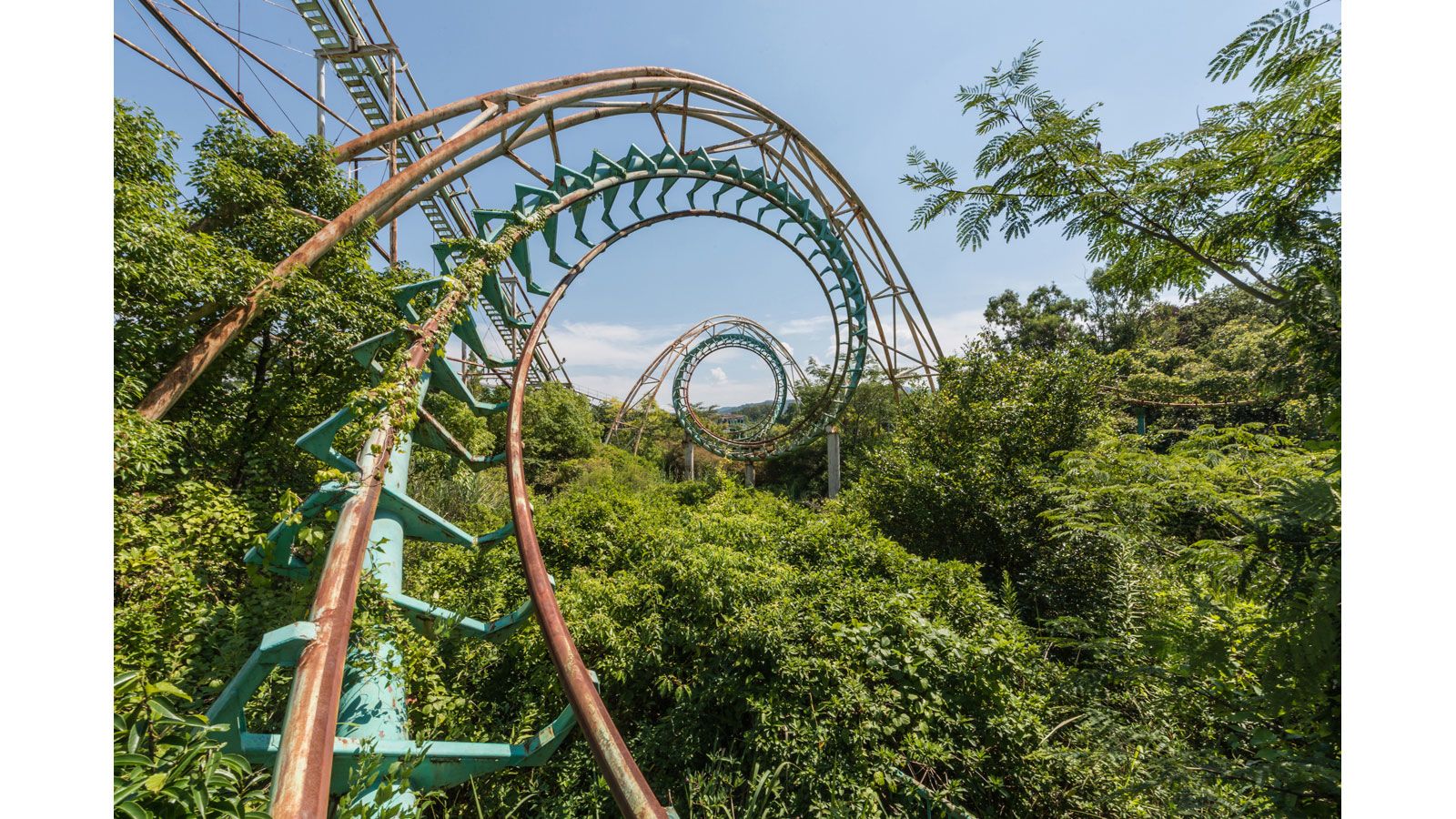This horizontal-rectangular image captures an intriguing and somewhat eerie countryside scene featuring an abandoned roller coaster cutting through a dense, overgrown forest. The perspective is a POV shot from the front seat of the coaster, with the track unrolling before the viewer. The roller coaster track, a teal hue with noticeably rusted light brown rails, starts from the bottom left and spirals into a series of tight loops at the center of the image, held up by metal supports that are greenish in color.

The track's abandonment is emphasized by the way large, overgrown trees encroach upon and even grow into the rails, making the scene appear unkempt and untamed. The sky above is a clear blue, occasionally dotted with distant clouds, offering a stark contrast to the chaotic scene below. 

Further up in the image, barely visible, is what seems to be an additional rail or perhaps a maintenance stairway, suggesting the vastness and complexity of the coaster structure. This added elevation emphasizes the sheer drop and height of the roller coaster, evoking a sense of thrill and peril.